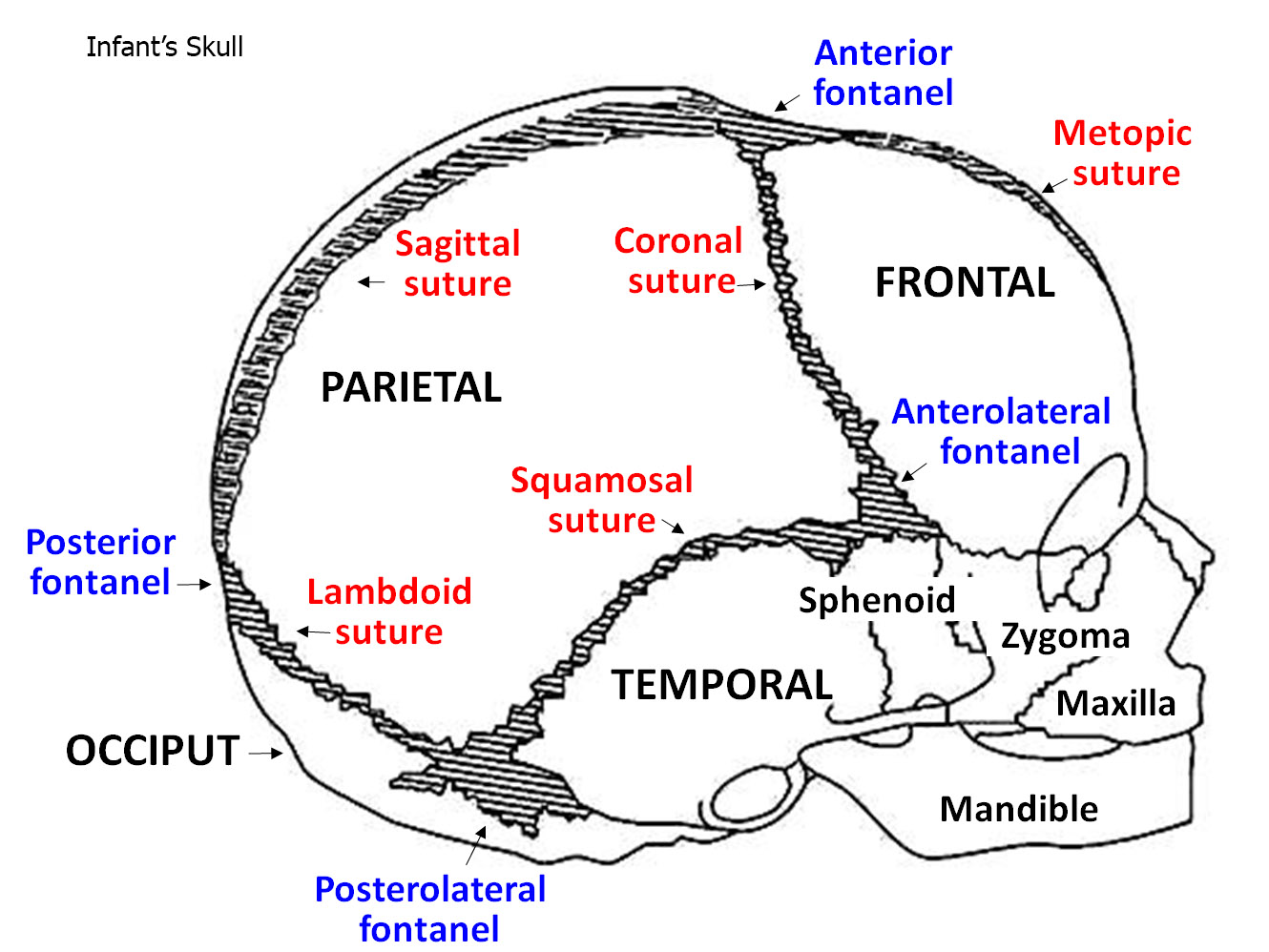This black-and-white sketch illustrates the intricacies of an infant's skull, highlighting the various sections and suture lines in detail. The skull, depicted facing to the right, is meticulously labeled with terms written in red, blue, and black ink. The frontal, parietal, occipital, temporal, and mandible bones are annotated, providing a comprehensive view of the cranial structure. Key sutures such as the coronal, sagittal, metopic, squamosal, and lambdoid are prominently marked in red. Additionally, the image identifies crucial fontanels: the anterior, anterolateral, posterolateral, and posterior, essential soft spots in an infant's skull. Labels in black ink point out further anatomical features including the sphenoid, zygomatic, maxilla, and cephaloid. This detailed illustration serves as an educational tool, showcasing the complex anatomy of an infant's skull without any surrounding flesh or blood, making the bone structures and connective sutures clearly visible.